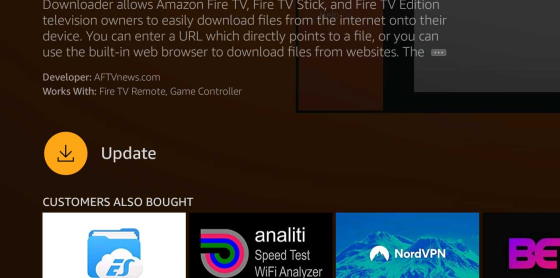The image features a black background showcasing promotional information about the "Downloader" app, specifically designed for Amazon Fire TV, Fire TV Stick, and Fire TV Edition televisions. In the center of the image, text explains that the Downloader app allows users to easily download files from the internet directly onto their device. Users can either enter a URL that points directly to a file or use the built-in web browser to download files from websites. 

Adjacent to the descriptive text, there is an emblem containing a 'V' and a small box with three stars in it, indicating a rating or feature highlight. Below this, it mentions the developer’s website, aftviews.com, and notes that the app is compatible with the Fire TV remote and game controller.

On the right side of the image, a miniature TV set graphic is present in the background. Below this, a yellow circle with a half box and a down arrow is labelled "Update," and a section titled "Customers Also Bought" follows. This section includes several app icons: a white box with a blue "ES" representing ES File Explorer, another icon for Anality Speed Test Wi-Fi Analyzer that features a gray, pink, blue, and green hook design, a blue box stating NordVPN, and a purple box with the letters "BE."